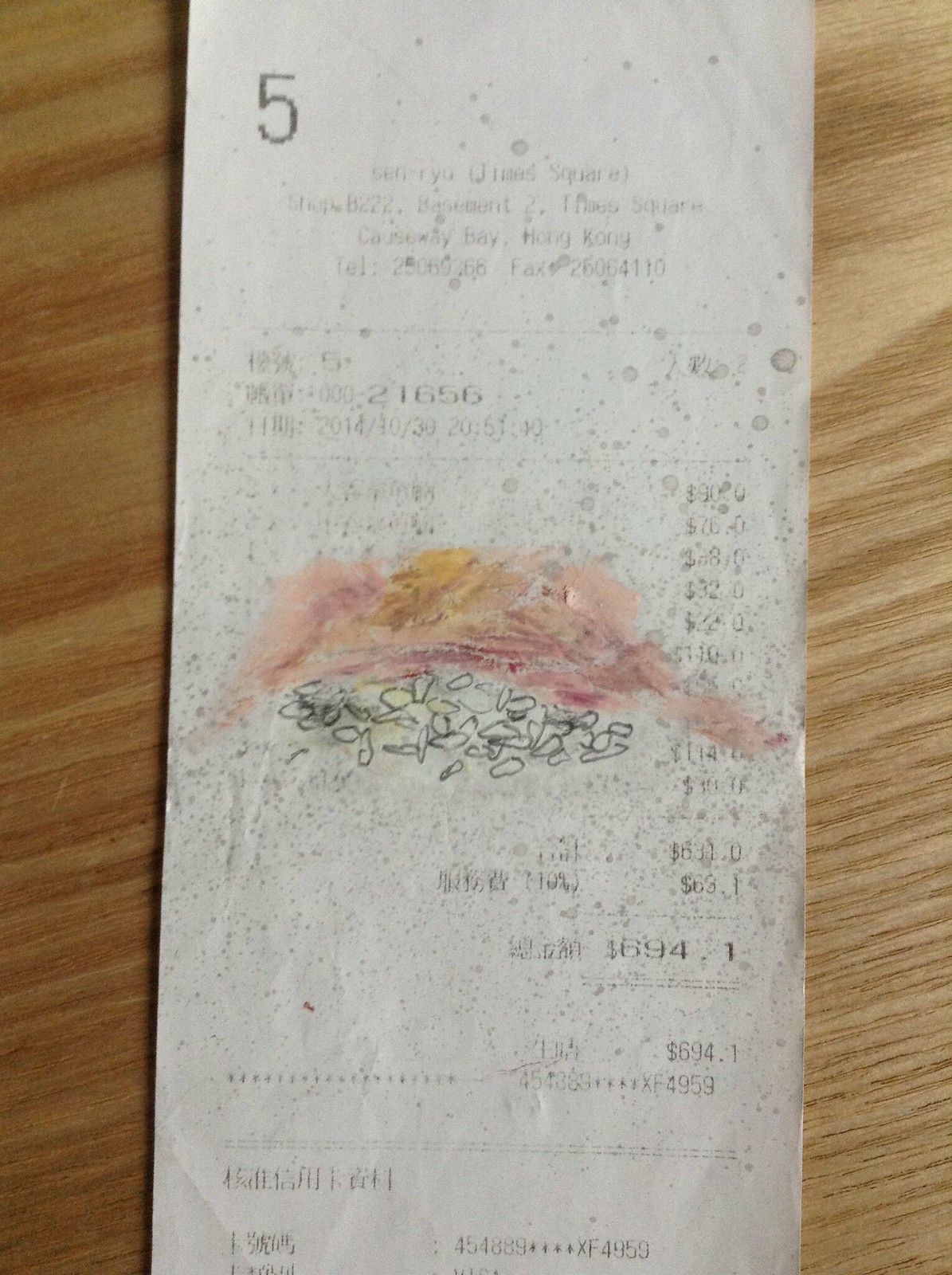A close-up photograph captures the entirety of an aged, worn receipt, positioned neatly at the center of the image against a rustic wooden table backdrop. The receipt, showing signs of wear and faded ink, displays several discernible elements despite its overall faded text. Dominantly featured is the number "5" and a total amount of $694.01 towards the lower section of the receipt, indicating a substantial transaction likely settled with a credit card. Adding an intriguing, personal touch, the receipt's center bears scribbles made with crayon and blackish pen, suggestive of spontaneous doodling or annotations. This juxtaposition of mundane financial documentation with whimsical markings creates a compelling visual narrative.